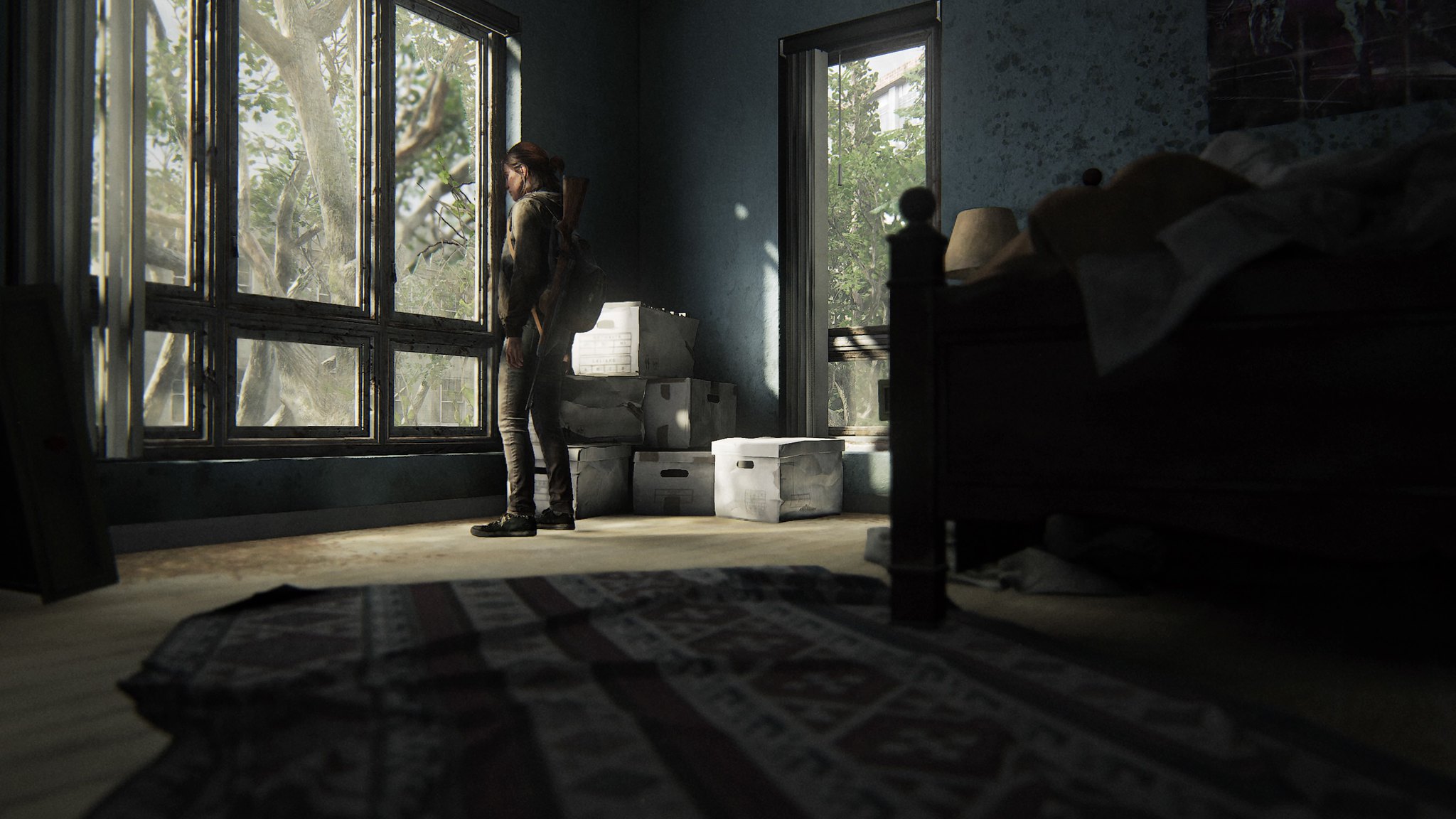In this image from a video game, we observe a detailed scene from the low vantage point of a bedroom floor. The room features a black and gray striped rug over light gray flooring. A character stands with their back to the viewer, dressed in gray pants, a gray sweatshirt, and a gray backpack, with the brown barrel of a shotgun visibly protruding. The character gazes out through a window, beyond which a series of trees with brown trunks and green leaves can be seen. To the left of the window hangs a light gray curtain. The bedroom's walls are painted gray, complementing a black bed frame positioned along one wall. In the corner to the right of the character, a stack of light gray boxes is visible, and to their far right, an open door reveals additional trees outside.